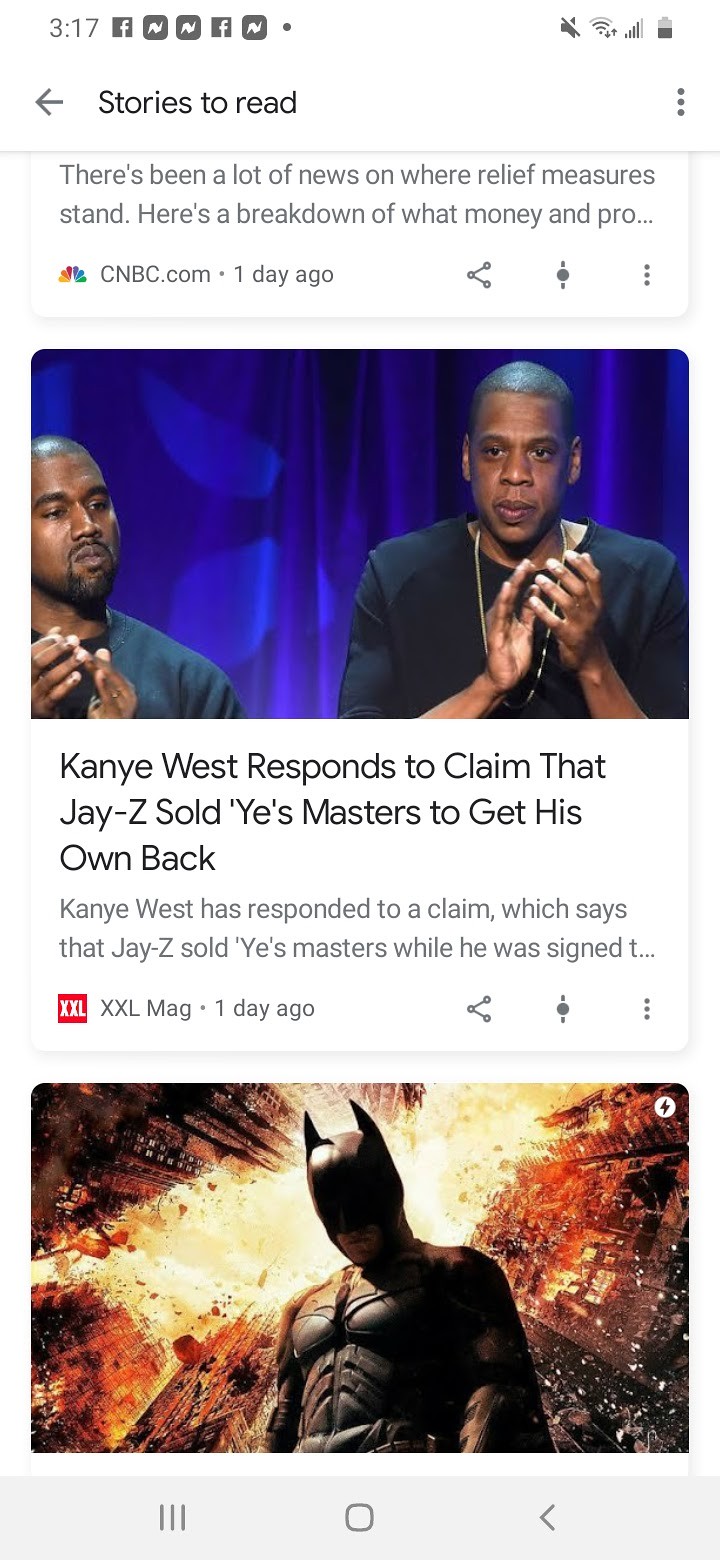The image depicts a vertically oriented social media feed displayed on a phone's screen at 3:17 PM. The top section of the screen includes an arrow pointing left, possibly indicating a back button, followed by "Your notifications" text, Wi-Fi, and battery icons showing half battery life and full Wi-Fi strength. The background is white, adorned with a few grey wavy line icons.

The first visible post in the feed, labeled from CNBC.com a day ago, discusses recent updates on relief measures, although the text cuts off after “Here’s a breakdown of what money and pro...”. Below this, a more prominent post displays an image of Kanye West and Jay-Z against a blue background, applauding on what appears to be a stage. The headline reads, "Kanye West responds to claim that Jay-Z sold Ye’s masters to get his own back," sourced from XXLmag a day ago.

Another section of the feed shows a shadowed image of Batman set against a fiery backdrop, suggesting an explosion or flames behind him. Batman’s face is dark, and his head is hung low, adding a dramatic tone to the scene. The overall feed likely belongs to Facebook given the icon repetition and layout.